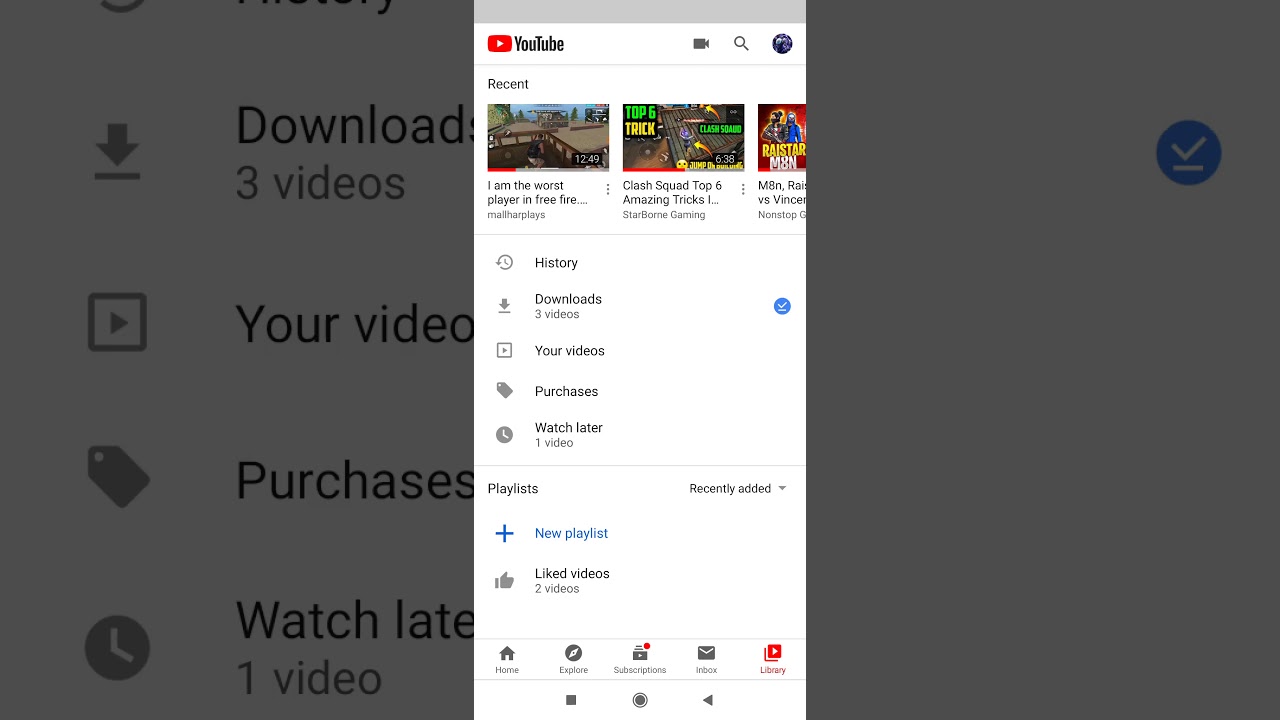The image is a screenshot from the YouTube website, showcasing the user interface for video management and viewing options. It prominently displays a vertical, elongated panel, listing three recent videos. The titles of these videos are: "I am the Worst Player in Free Fire," "Clash Squad Top and Amazing Tricks," and another with an unreadable title, which features a red thumbnail with people underneath.

Above these listings is a section labeled 'History,' which shows 'Downloads,' 'Three Videos,' 'Your Videos,' 'Purchases,' and 'Watch Later - One Video.' On the right side of this section, there is a blue circle with a white checkmark. Below this, there is a heading that says 'Playlist Recently Added,' followed by 'New Playlist' in blue with a blue plus sign next to it. Additional entries include 'Liked Videos - Two Videos' with a thumbs-up icon next to it.

At the bottom of the page, there are several icons indicating navigation options: a home icon, an explore icon, and a few others that are partially obscured. One of the icons is a box with a red circle next to it, another is an envelope, and there is a red box with a white arrow pointing to the right.

This YouTube interface is overlaid on another website, which also shows part of the same information: 'Downloads,' 'Three Videos,' 'Your Videos,' 'Purchases,' and 'Watch Later - One Video,' duplicated in a white, blurred background.